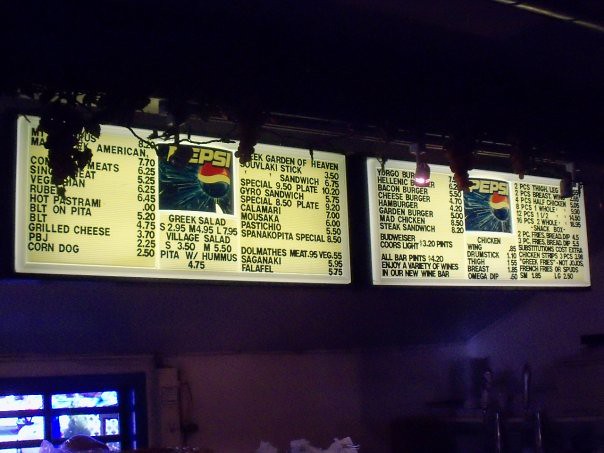The image depicts a brightly-lit menu board in an electrical fast food setting, illuminated by overhead lights. The board itself is predominantly white with red lettering, detailing various fast food items and their prices. Prices are positioned to the left of the food items listed on the right. 

Prominently displayed on the board is a Pepsi logo, featuring the brand's signature red, white, and blue swirl on a bluish background, giving a sense of motion with white light streaks. 

The backdrop of the image is a dark, almost purple hue. There is a black-framed window with intricate inner frames adding to the overall composition.

Menu items are listed as follows:
- Left bottom: Corndog - $2.50, above that PBJ - $2.25, Grilled Cheese - $3.70, BLT - $4.75, BLT on Pita - $5.20.
- Below the Pepsi sign on the left: Greek Salad (Small - $2.95, Medium - $4.95, Large - $7.95), Village Salad (Small - $3.50, Medium - $5.50), Pita with Hummus - $4.75.

Other similar fast food items and prices fill the rest of the board, albeit some parts are slightly blurry.